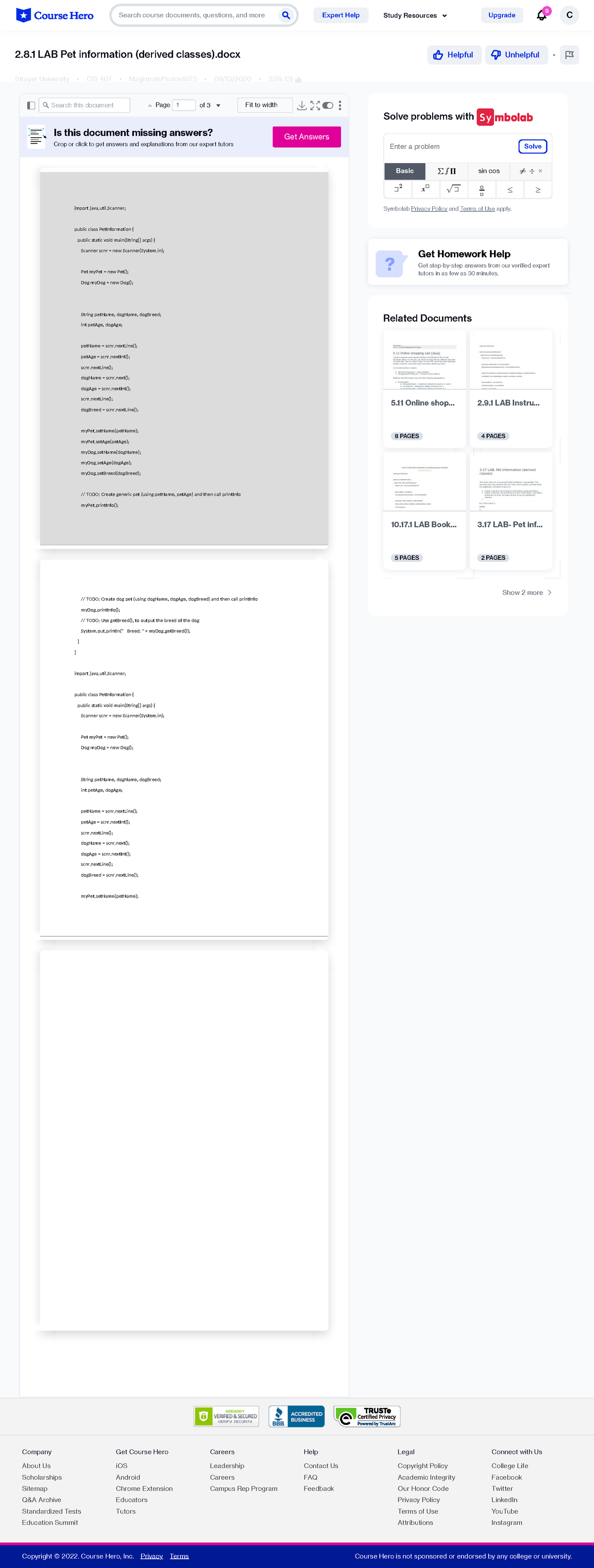This image displays a comprehensive view of a website page, perfectly fitting within the screen without requiring any scrolling. The layout is rectangular, reminiscent of a mobile screenshot but displayed fully on one flat plane.

At the top left, there is a distinctive blue company logo, followed closely to the right by a search bar. Adjacent to the search bar is a large gray button, and to the left of this button, there is a dropdown box with small black text.

On the left side of the page, there is a document form showcasing three full pages, which are vertically arranged. The first page is grayed out, while the other two are in white. Above the first page, there is an array of dropdown menus and text box options. Specifically, there is one text box option to the far left, followed by two additional text box options to the right, and a section for changing the font. Further right, there are three small boxes. The top-right box features characters with categories labeled above it, and the first category is currently selected. A red logo is visible at the top right corner of the first white box.

Below this section is a rectangular box containing a blue icon on the left and bold black text on the right. Underneath, there is a section featuring four document thumbnails with a "Recent Documents" label positioned at the top left of the box.

The footer at the bottom of the screenshot includes three centered icons, likely representing affiliations such as the Better Business Bureau. Below the icons, categories are listed vertically down the page.